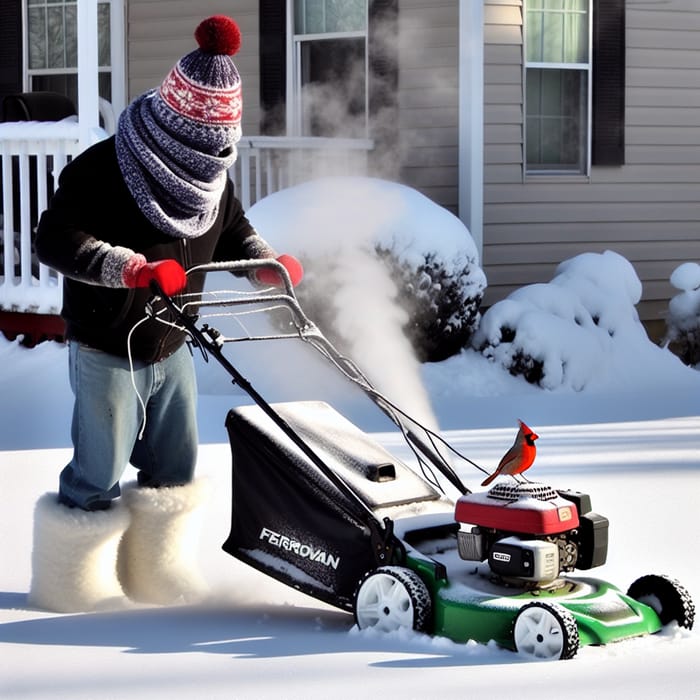In this whimsical winter scene, a person is using a green snowblower, disguised to look like a lawnmower, to clear the snow off the walkway of a brown house with black shutters and snow-covered bushes. The person is bundled up in a black long-sleeve jacket, jeans, and large, fluffy white wool boots that seem un-waterproofed. Their face is completely wrapped in a thick wool scarf, topped with a grey knitted hat featuring a red stripe and a red pom-pom, and they have red gloves on their hands. The motor of the snowblower is red, and, charmingly perched on it, is a vibrant red cardinal. There are no tracks behind the snowblower, indicating it has just started. The scene's enchanting strangeness, combined with the harmonious elements of winter attire and the playful presence of the cardinal, adds a touch of magic, making it feel almost surreal or AI-generated.